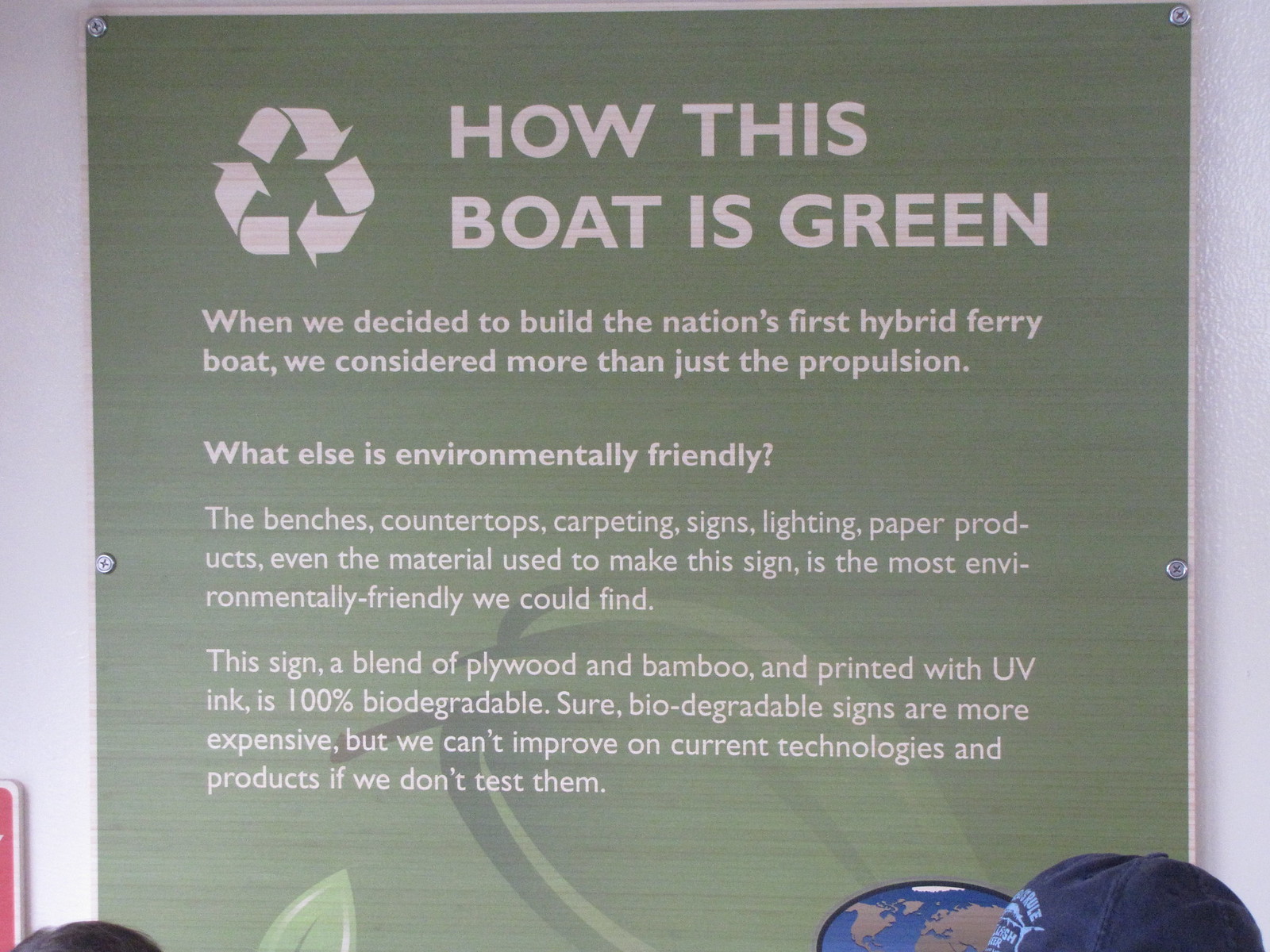The image shows a green sideboard mounted on a white wall, secured with four metal pins—two at the top corners and two at the middle sides of the board. The sideboard features white text that explains the eco-friendly attributes of a hybrid ferry boat. At the top left, there's a white recycling logo consisting of three arrows forming a triangle. The main text begins with "How This Boat Is Green" in capital letters and continues to outline that when building the nation's first hybrid ferry, considerations extended beyond propulsion to include benches, countertops, carpeting, lighting, and other materials. Emphasizing sustainability, the sign mentions that even the sideboard itself is an eco-friendly blend of plywood and bamboo, printed with UV ink and is 100% biodegradable. Additional text elaborates on the importance of testing new technologies despite higher costs. The scene appears to be indoors, possibly during a presentation, with the heads and hats of a couple of people visible at the bottom corners of the image.